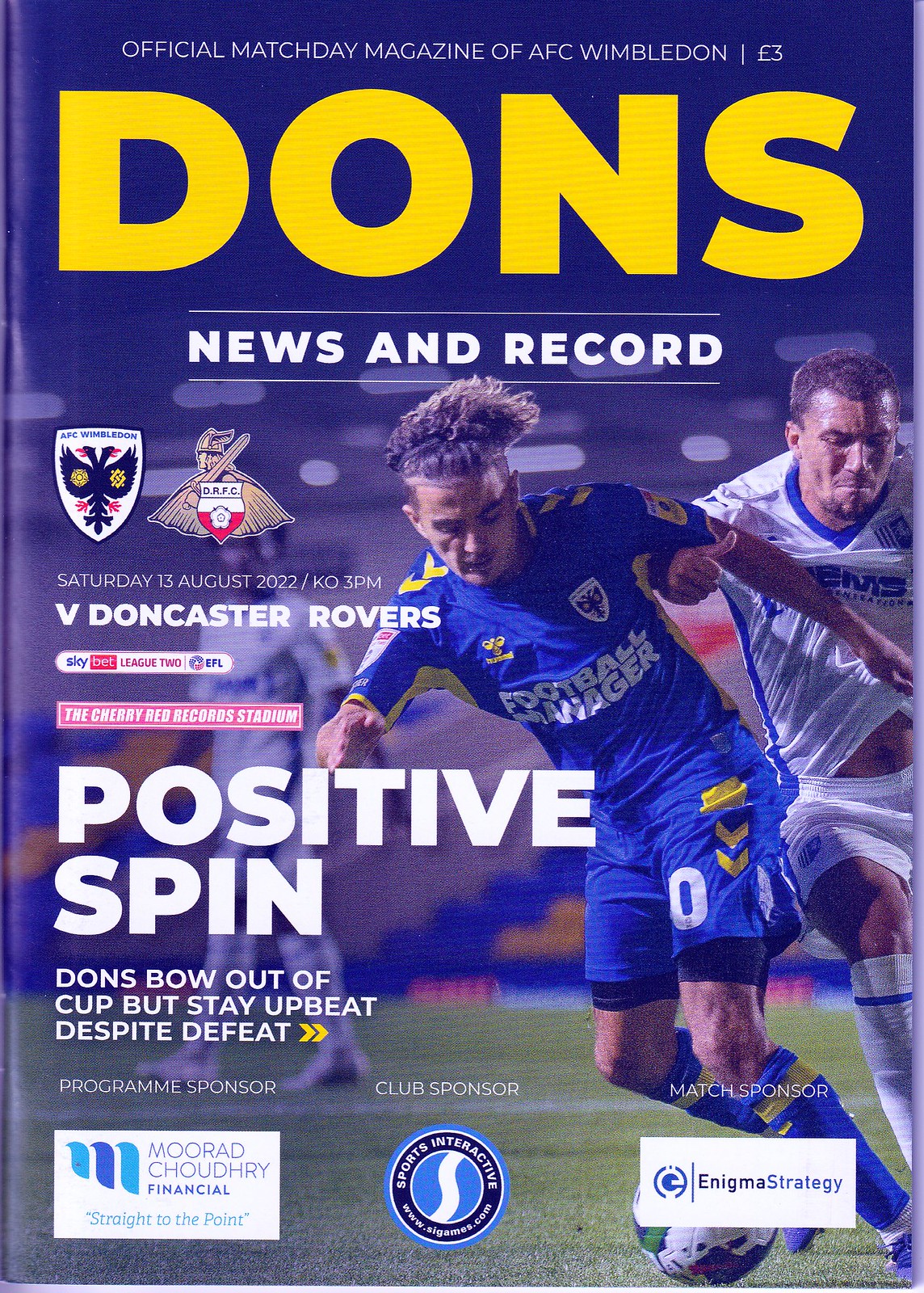This magazine cover features a predominantly blue background and is vertically oriented. At the top, bold yellow letters spell out "DONS," with smaller white text above reading "OFFICIAL MATCH DAY MAGAZINE OF AFC WIMBLEDON" and the price at £3. Underneath "DONS," white text in all caps reads "NEWS AND RECORD." 

On the right side of the cover, there is an action shot of two soccer players vying for the ball on the ground. The player on the left, wearing a wrinkled blue and yellow uniform with the partially visible text "FOOTBALL" and ending in "A-G-E-R," has tall, curly brown hair and blue shorts numbered "0." The player on the right is dressed in a white jersey and shorts, with short brown hair.

To the left, adjacent to the title, is the AFC Wimbledon logo featuring a double-headed bird with yellow insignias on its wings. Next to it is a smaller logo depicting a knight with a cape and a shield labeled "D.R.F.C." Below these logos, text reads "SATURDAY 13TH AUGUST 2022, K.O. 3PM, V. DONCASTER ROVERS" in a mixture of standard and bold white text.

Further down, a red rectangular box contains the text "THE CHERRY RED RECORDS STADIUM." Large white capital letters below this announce "POSITIVE SPIN," followed by "DONS BOW OUT OF CUP BUT STAY UPBEAT DESPITE DEFEAT." 

At the bottom, advertisements for "MURAD CHAUDHRY FINANCIAL," "SPORTS INTERACTIVE," and "ENIGMA STRATEGY" appear alongside the Sky League 2 logo.